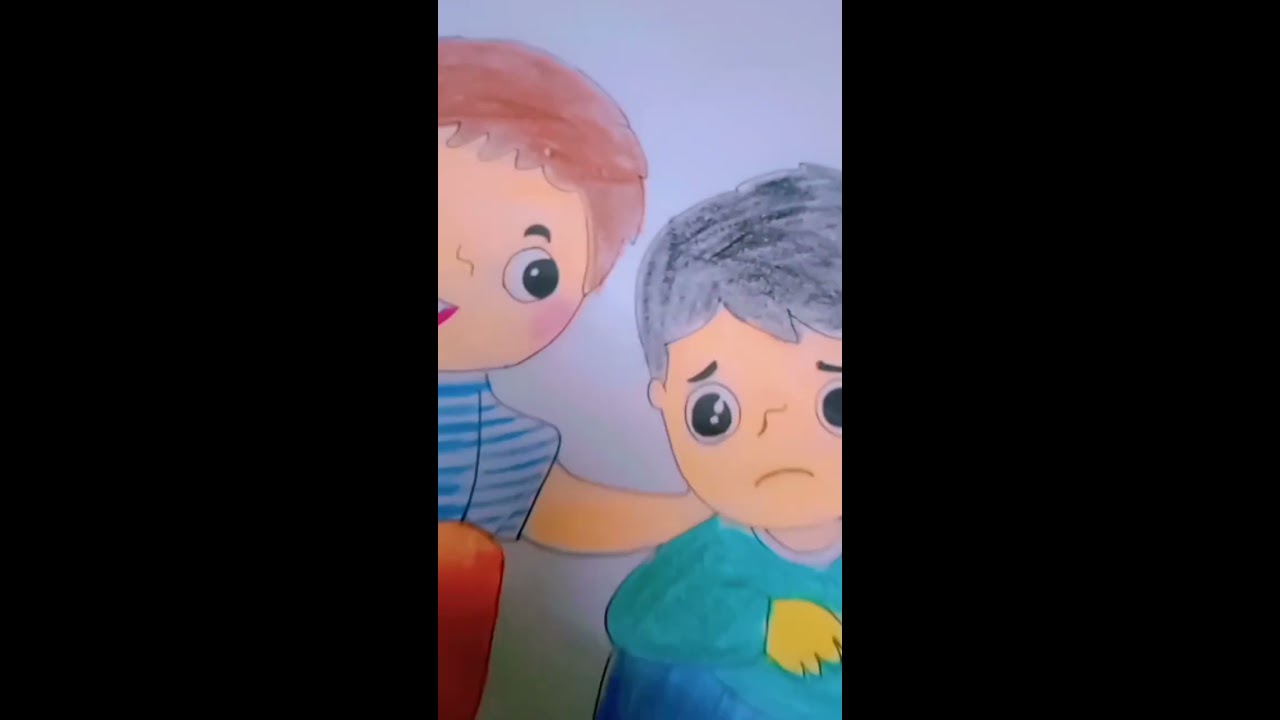This vibrant, marker or paint-drawn illustration showcases two children set against a very light blue, nearly white background. The scene captures a touching moment of comfort, as the child on the left with brownish-red hair, large circular eyes, and a blue striped shirt paired with orange pants, reaches out with his left arm to console his friend. The consoling child, visible only partially due to a prominent black border framing the image, has a sympathetic expression with a hint of a smile. The boy on the right, depicted in a teal green shirt and jeans, has dark hair and large, sorrowful eyes. His downturned mouth and slanted eyebrows clearly express sadness, as he sits or slouches slightly, feeling the comforting hand of his friend on his shoulder. The wide black borders on either side suggest a cropped or focused view, emphasizing the emotional interaction between the two figures.